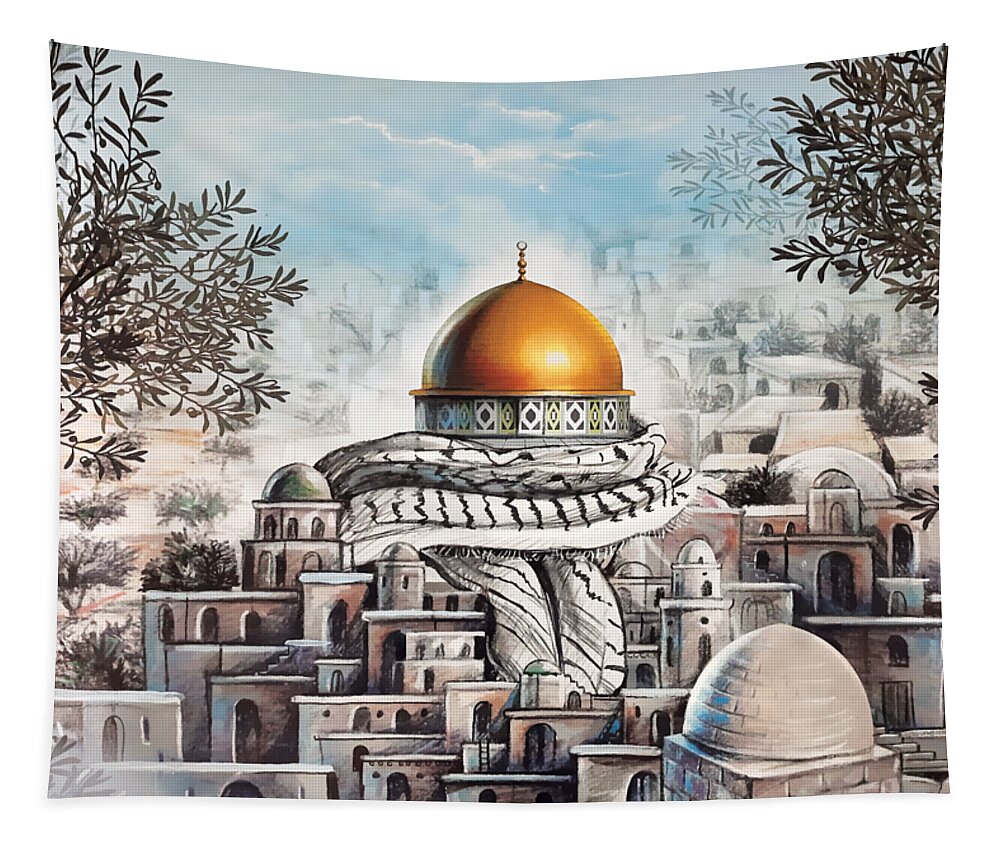This image is an artistic rendering, likely painted on cloth or resembling a tapestry, depicting a vibrant cityscape. At the center is a towering building crowned by a large, radiant orange-gold dome reminiscent of the Dome of the Rock in Jerusalem. This striking dome features stacked gold orbs topped with a golden ring and is adorned with intricate diamond-shaped patterns. Notably, a black and white striped scarf wraps around the dome's base, extending over some of the surrounding smaller buildings.

The city stretches across a hillside, characterized by white homes with large, dark arched doorways, creating a picturesque postcard-style Moroccan village. The buildings, appearing as if stacked upon one another, spread throughout the foreground and blend seamlessly into the background. Olive tree-like foliage is visible on the left side, adding to the lush scenery.

Above, a slightly hazy blue sky is dotted with puffy white clouds. Green branches from deciduous trees frame both sides of the image, adding depth and enhancing the dynamic composition of this detailed cityscape.